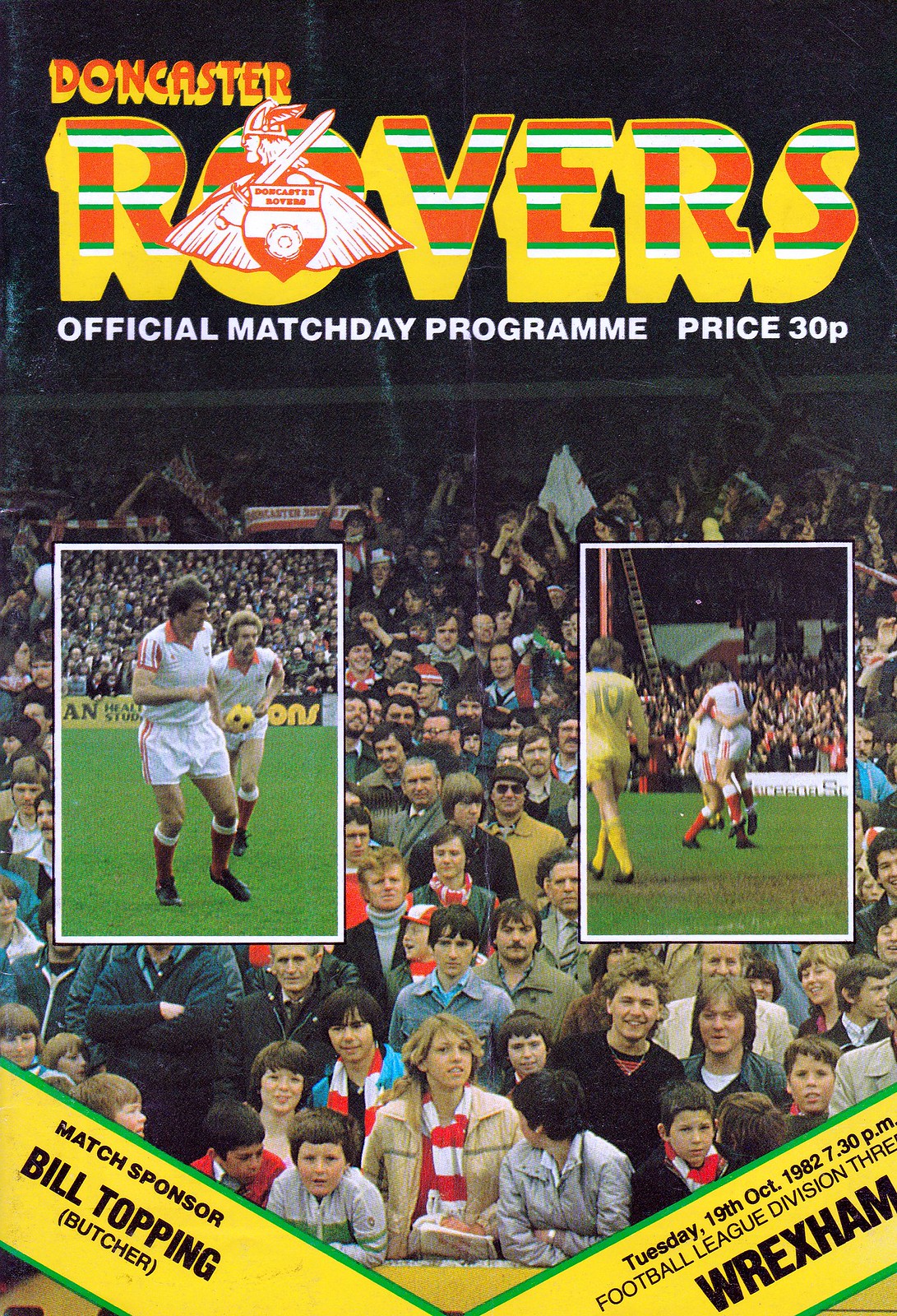The image is a magazine cover: the official match day program for the Doncaster Rovers, priced at 30p. Dominating the background is a vibrant photo of a crowded stadium, brimming with spectators. Overlaying this crowd scene are two smaller action shots of soccer players, who are seen in dynamic poses, showcasing the excitement of the game. The top of the cover features the title "Doncaster Rovers" in a striking 3D font with hues of orange, yellow, green, and white. Embedded within the ‘O’ of "Rovers" is the Doncaster Rovers crest, depicting a Viking carrying a sword and shield. Below the title, in smaller white text, it reads "Official Match Day Program". At the bottom corners of the cover, there are yellow banners with green borders. The left banner indicates the match sponsor, "Bill Topping Butcher," while the right details the match information: "Tuesday, 19th October 1982, 7:30 p.m., Football League Division 3, against Wrexham."